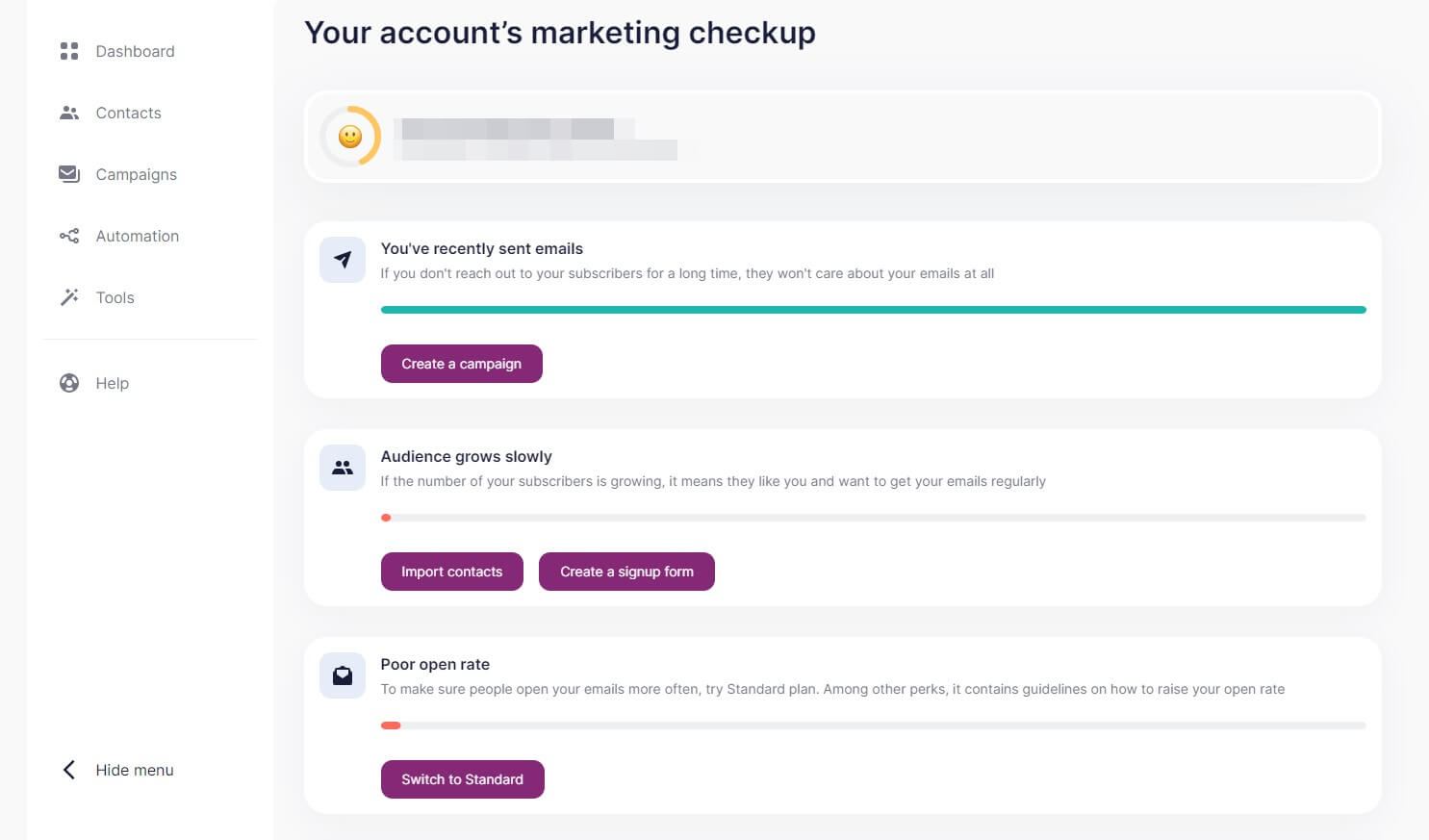This image displays a screenshot of a website's dashboard page, designed with a user-friendly interface. 

On the left side, a white sidebar lists six navigational options, each accompanied by an icon on the left and text on the right. The options are labeled as follows: Dashboard, Contacts, Campaigns, Automation, Tools, and Help. At the bottom of this sidebar, there is an option to "Hide Menu," featuring a back arrow icon to the left.

The main content on the right starts at the top with the heading "Your Account's Marketing Checkup." Below this heading, there is a prominent circular progress bar with a smiley face icon inside it, indicating an overall status or health check of the account. Adjacent to this graphic, on the right, is a blurred section containing obscured information, likely specific account details.

Beneath this section, three white boxes are aligned horizontally, each focusing on different aspects of the account's performance. These sections are:

1. "You've Recently Sent Emails" – This section might contain a summary or details about the latest email campaigns sent.
2. "Audience Grows Slowly" – This box presumably addresses the rate of audience growth, with an indication of areas needing improvement.
3. "Poor Open Rate" – This section highlights email open rates, pointing out concerns regarding engagement levels.

Each of these sections is titled at the top, features an icon on the left, and includes a purple button at the bottom, likely providing options for further actions or more detailed insights.